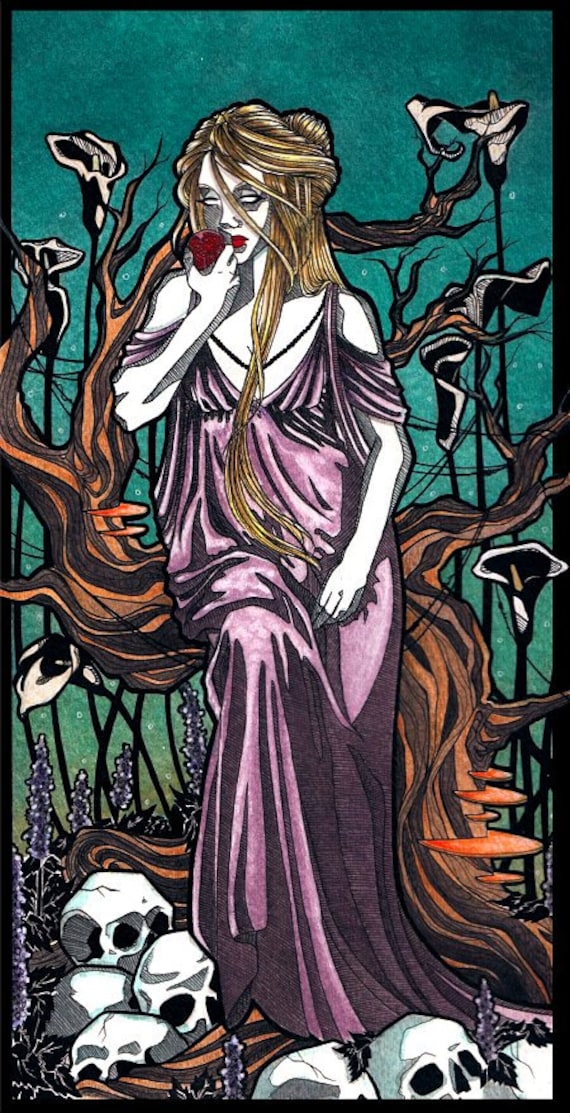This artwork features a haunting image of a woman with long, flowing blonde hair styled in a bun, wearing a long purple dress. Her eyes, stark white and pupil-less, add to the eerie atmosphere of the piece. She sits on the irregular branches of a lifeless tree, surrounded by tall, thin flowers that resemble corpse lilies, primarily white with hints of yellow. At her feet lie several white skulls, symbolizing death. The background is a mix of blue and green hues, enhancing the otherworldly, almost comic book-like quality of the scene. In her hand, she holds a red apple close to her lips, hinting at a deeper, possibly sinister narrative.